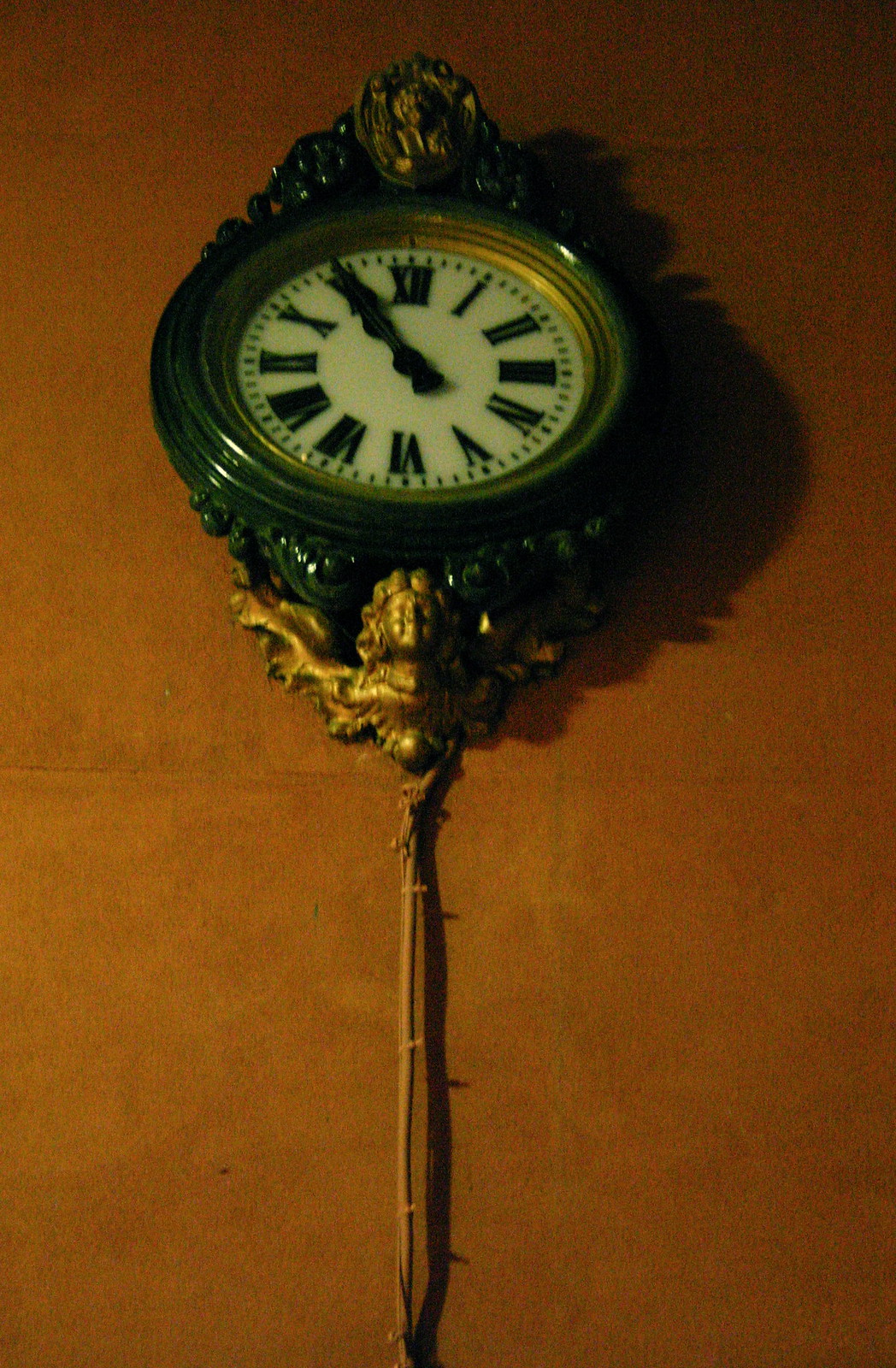This is a color photograph of an ornate, antique-looking wall clock. The clock face is white with black Roman numerals arranged from I to XII, indicating the time, which is approximately 10:50 or 10:55, as both hands point near the XI. The clock's exterior features a bronze or dark green color, giving it an old-school appearance. Mounted on a brownish-red wall, possibly made of larger bricks or panels, the clock also casts a prominent shadow to the right due to the dim lighting in the area. 

Adding to its ornate detail, there's an emblem above the clock face that resembles a lion's head, while the bottom boasts a darker gold, sculpted figure of a cherub or a woman's head and chest, which appears to be supporting the clock. A decorative yellow pendulum string hangs below the clock, though it does not seem to serve any functional purpose, adding to the antique aesthetic of the piece.